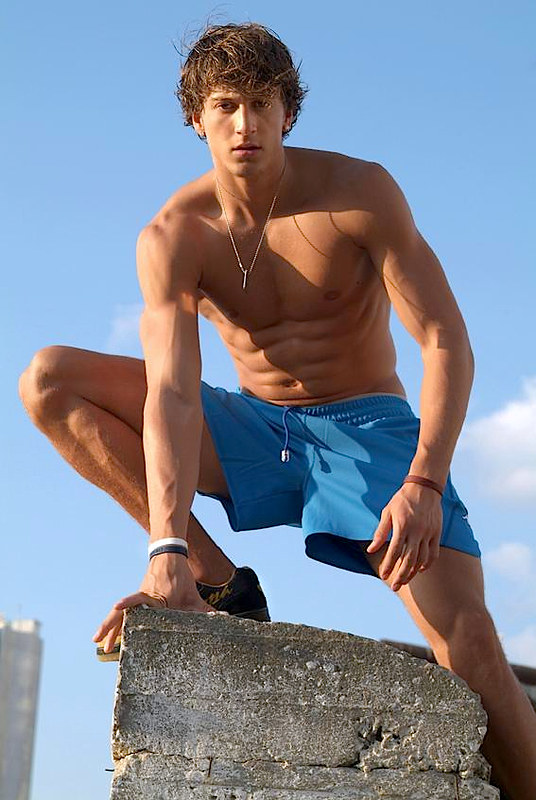The image features a young, tanned man in his early twenties with a surfer aesthetic. His medium-length, brown hair appears wet, suggesting a beach setting under sunny and warm weather. He is wearing a short blue bathing suit with a distinctive drawstring capped by a clear end, and black shoes that resemble Vans. He sports a silver necklace with a pendant that has the feel of a dog tag. Additionally, he has wristbands on both wrists—one light yellow, one dark blue, and another brown. The young man, who has a lean yet muscular build with defined abs, is posing on a crumbling stone wall, one leg up, staring directly into the camera. The background is a vast, clear sky with a touch of cloud on the right. This composition, along with his model-like pose, highlights his confident demeanor.